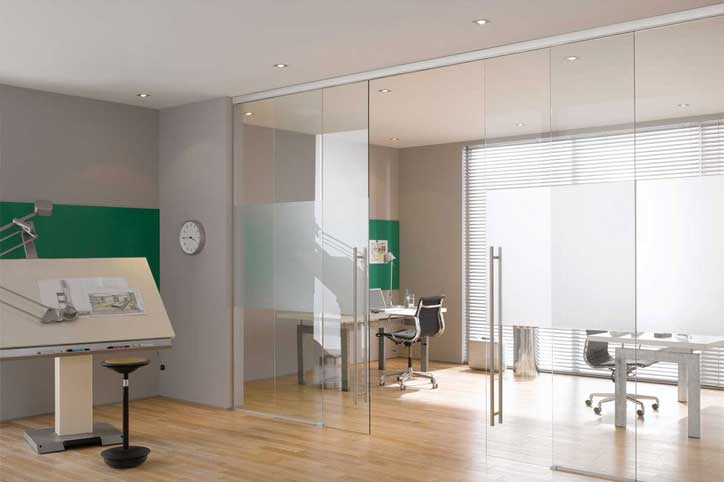The photograph showcases the interior of a contemporary office, featuring a stylish and open layout. Central to the image is a spacious room with floor-to-ceiling glass walls, including a large sliding double door that is currently open. The center of the glass door is frosted to prevent accidental collisions, enhancing both safety and aesthetics. Inside the glass-walled room, two wooden desks, each accompanied by a chair, are situated side by side. This workspace is bathed in natural light, thanks to the large, shaded windows lining the right-hand wall.

On the left side of the image, there is a well-equipped design area, possibly for architectural work, which includes a large drafting table and a stool. Adjacent to this design space is a green board, adding a pop of color and functionality to the room. The interior room also features a small podium or standing desk with some papers on it.

Both rooms share a seamless light wooden floor, and the walls are painted a sleek gray, contrasted by a white ceiling. A clock adorns one of the walls, reinforcing the professional atmosphere of the space. Overall, the detailed layout and specialized furnishings suggest this office serves as a creative workspace, possibly for architects or designers.